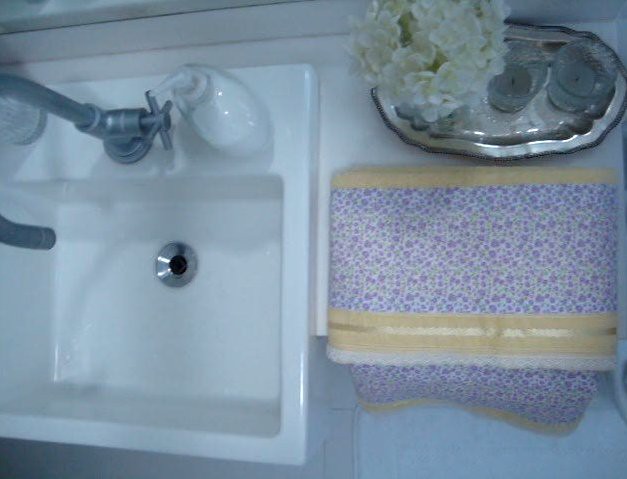This photograph provides a bird's-eye view of a meticulously arranged bathroom sink setup. The sink is a surface-mounted, white porcelain square fixture with a slightly protruding edge. A high arch pewter silver faucet with a single knob, indicating the water is at an optimal temperature, is centrally positioned. To the right of the faucet stands a glass pump bottle, while to the left, the base of a clear glass is visible. The drain opening is a gleaming stainless steel, adding a touch of elegance to the sink.

Adjacent to the sink on the right side, a sophisticated silver tray is showcased. The tray holds two pink candles, a small bouquet of cream-colored artificial flowers, and a neatly folded towel. The towel is adorned with a delicate pattern of purple or lavender flowers on a white background, finished with a luxurious tan edging and a shiny gold stripe.

In the foreground, the floor beneath the sink area is visible, featuring a plush fleece mat that adds comfort and style to the bathroom space. This well-composed scene captures the essence of a serene and elegant bathroom.